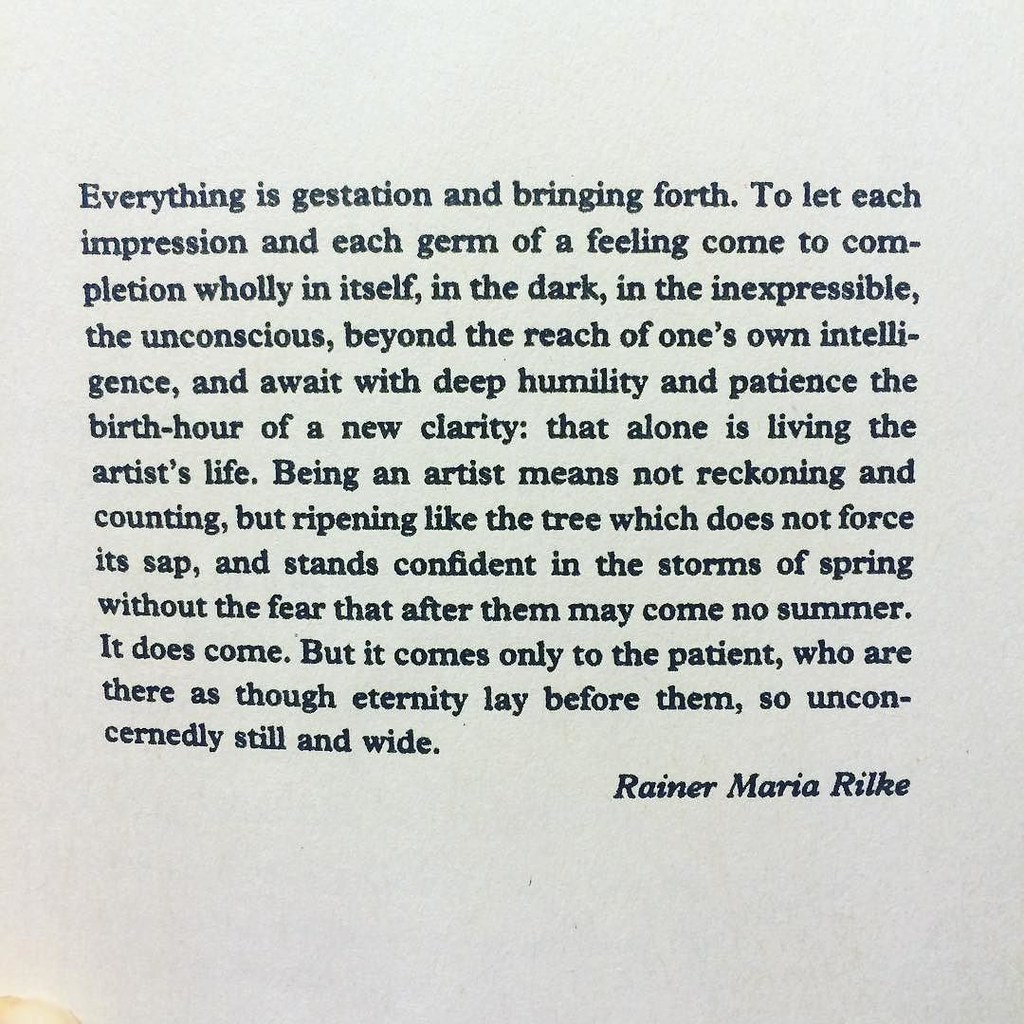This is a close-up image of an excerpt from a book, featuring a quote by Rainer Maria Rilke, printed in black font on white paper. The passage reads: "What is gestation and bringing forth? To let each impression and each germ of a feeling come to completion wholly in itself, in the dark, in the inexpressible, the unconscious, beyond the reach of one's own intelligence, and await with deep humility and patience the birth hour of a new clarity that alone is living the artist's life. Being an artist means not reckoning and counting, but ripening like the tree which does not force its sap and stands confident in the storms of spring without the fear that after them may come no summer. It does come, but it comes only to the patient who are there as though eternity lay before them, so unconcernedly still and wide." In the bottom right corner, the author's name, Rainer Maria Rilke, is clearly visible. Adding a touch of character, a small coffee stain is noticeable in the bottom left corner of the page.